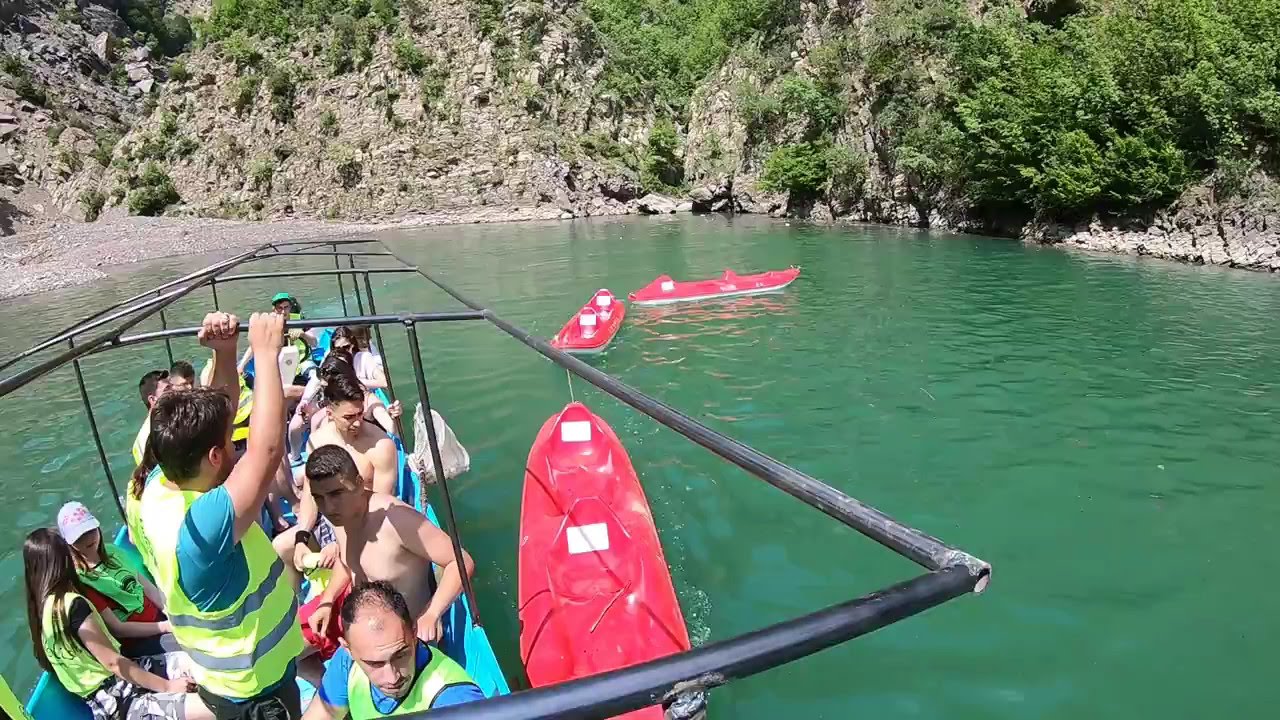The photograph captures a group of approximately 15 young people tightly packed on a narrow, blue, rectangular boat. The boat, featuring a prominent black metal frame at the top as if meant to support a canopy, occupies the bottom left corner of the image. Most of the individuals are wearing yellow reflective vests, though some men are shirtless, contributing to the diverse attire depicted. Adjacent to the boat on the right, three red, two-seater paddle boats or kayaks are tied together in a line. The background reveals a serene cove with still, medium-toned green water, surrounded by rocky cliffs adorned with patches of green bushes. This setting, with its defined cliffs and tranquil water, encapsulates a peaceful yet active scene on the water.